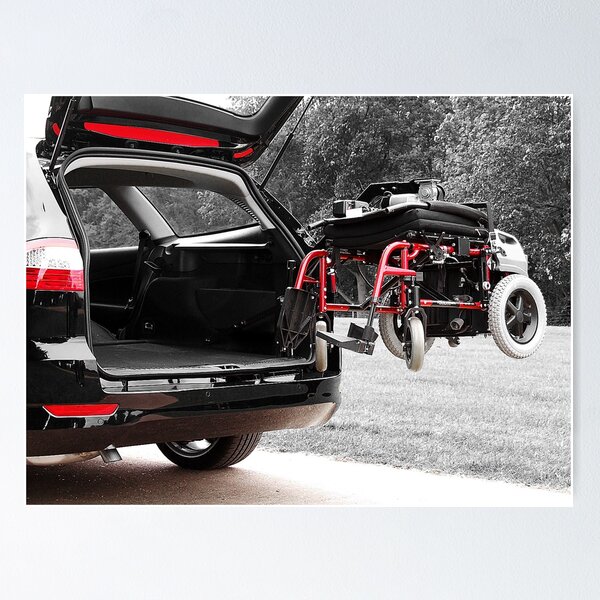The black-and-white photograph showcases the rear of an SUV or van on the left, with its back hatch fully open. At the center, a folded wheelchair is suspended mid-air, seemingly being hoisted by the vehicle. The wheelchair features prominently in the image, with a black seat and red metal bars forming its frame. The chair includes two smaller wheels at the front and two larger white wheels at the rear. The wheelchair appears to be designed for easy insertion or removal from the vehicle, which has its interior visible behind the raised hatch. One red and white brake light is evident on the left side of the vehicle. The backdrop consists of a gray sky, dark trees primarily on the right, and a light gray grass field extending across the background. Further details include a silver foot pedal on the wheelchair and the concrete surface beneath the van, adding to the monochromatic aesthetic punctuated by the striking red elements of the wheelchair and the brake light.